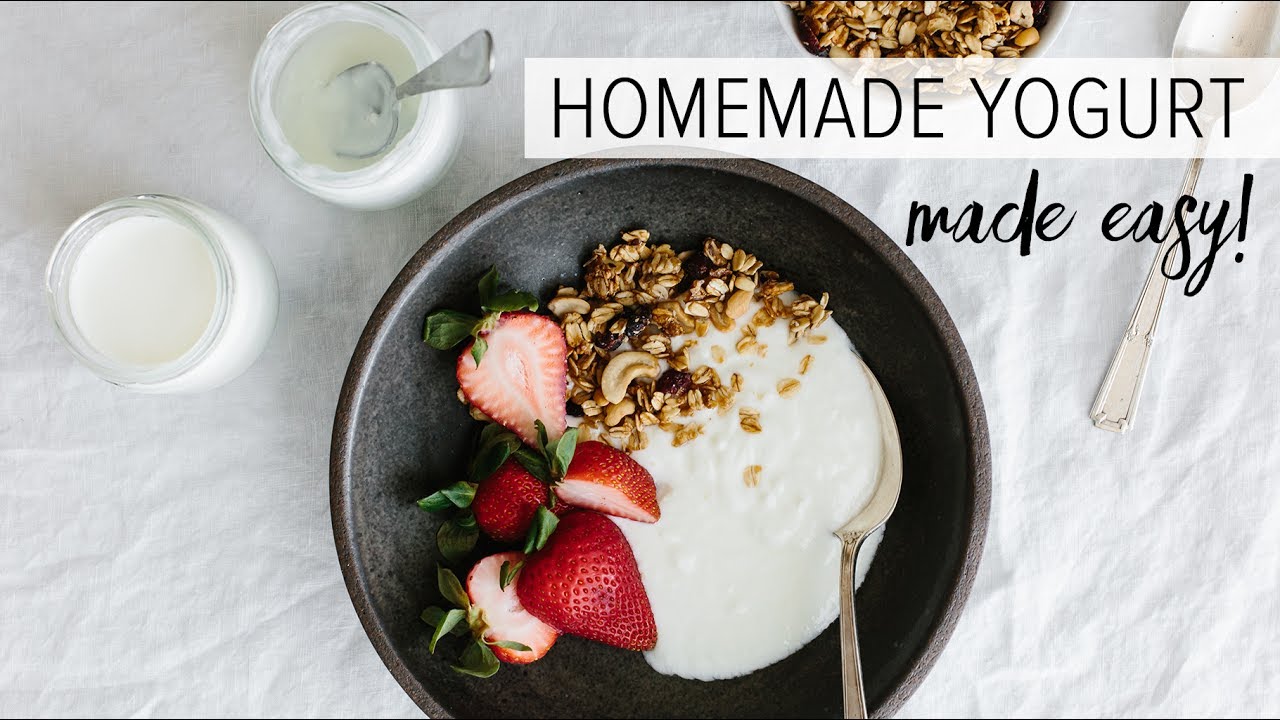This overhead photograph showcases an inviting spread for homemade yogurt on a white cloth background. At the center of the image is a black saucer containing Greek yogurt, elegantly arranged with a sprinkling of brown granola, and accompanied by vibrant, sliced strawberries and cherries on the left side. In the top left section of the image, two jars of yogurt are featured; one with a spoon inserted, indicating it has been used, while the other remains completely full. Adjacent to these jars is a smaller bowl of dry oatmeal. Towards the top right, a spoon lies face-up, its handle extending downwards and to the left. A white banner with bold, black text reads "Homemade Yogurt," and beneath it, in cursive writing, the phrase "Made Easy!" is displayed. This detailed setup appears to illustrate the simplicity and enjoyment of making one's own yogurt.